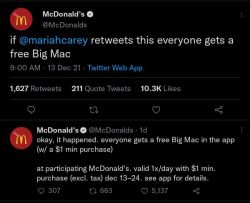This image is a screenshot captured from McDonald's official Twitter account, showcasing a promotional tweet on a black background. In the upper left corner, a red circle prominently features the iconic yellow McDonald's arch. To its right, "McDonald's" is displayed in bold white text, accompanied by a verified check mark and the handle "@McDonalds".

The highlighted tweet reads: "If @MariahCarey retweets this, everyone gets a free Big Mac." This message, tagged in blue with Mariah Carey's handle, was posted at 9:00 AM on December 13th, 2021, via Twitter Web App. Below this tweet, social metrics are visible—1627 retweets, 211 quote tweets, and 10.3 thousand likes. Icons for like, retweet, comment, and share are also displayed.

Beneath the initial tweet, McDonald's further responds: "Okay, it happened. Everyone gets a free Big Mac in the app (with a $1 minimum purchase at participating McDonald’s, 1x/day excluding tax, December 13th through 24th). See app for details." This follow-up includes the same red circle icon and text formatting, clarifying the offer's conditions.